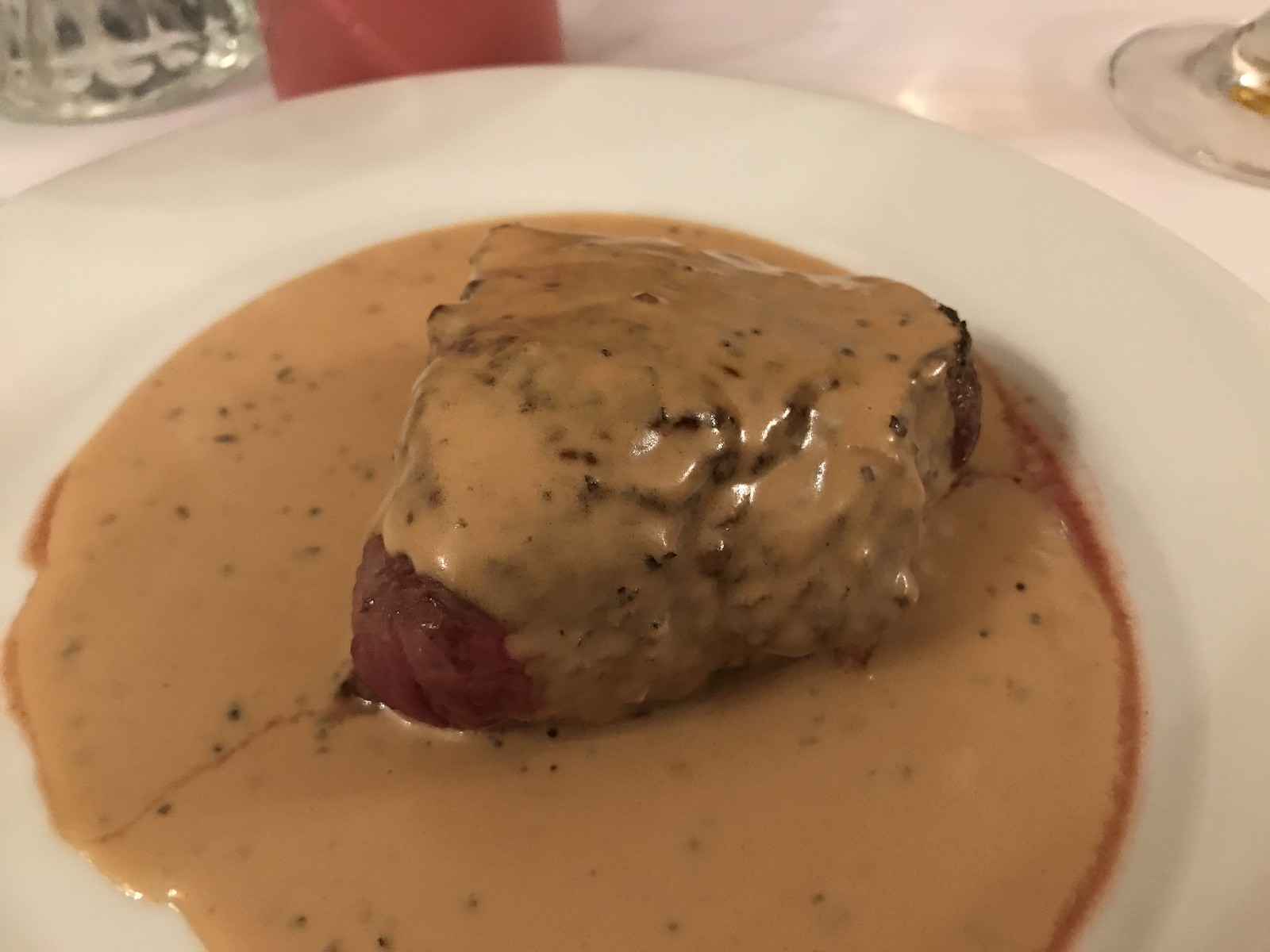The image showcases a white plate on a white tablecloth, holding a piece of brown meat or potentially a potato, generously coated in a light brown gravy that has formed a puddle on the plate. The gravy is speckled with small brown or black ingredients, possibly seasoning or pepper. In the background, there is a reddish pink drink towards the top of the picture, along with two glasses—one in the upper left corner and the base of another in the upper right. There is also another container placed between the two glasses. An overhead light source illuminates the scene, emphasizing the fine details of the food and the arrangement on the table, which does not include any dining utensils.